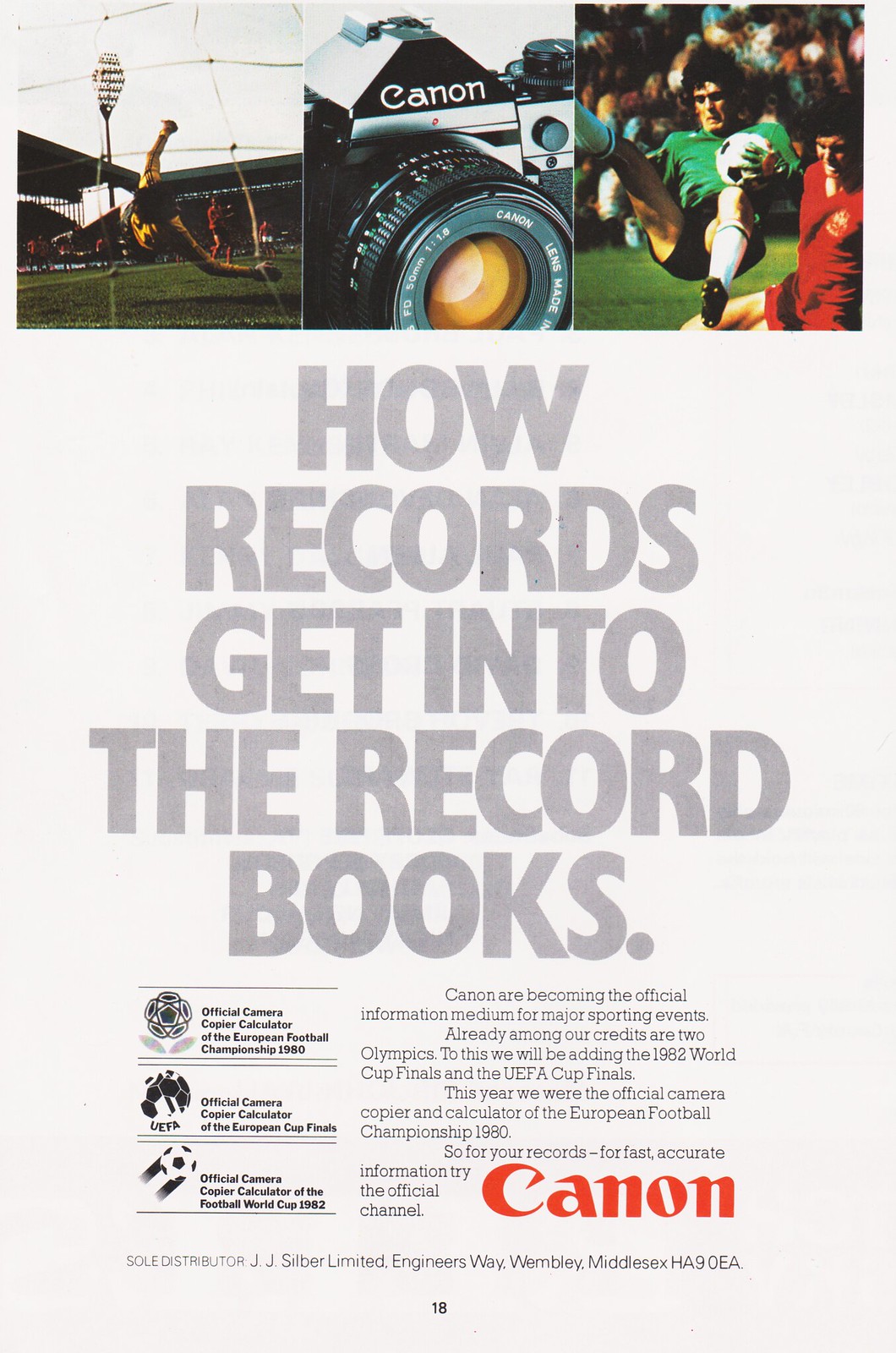This image is an advertisement for Canon, meticulously arranged with a compelling visual narrative and detailed promotional information. At the top, three dynamic photographs are aligned side by side. The first image depicts a soccer goalie in a dramatic mid-air save, captured from behind the goal's net. The middle image showcases a sleek, black Canon camera with a long lens, featuring a distinctive yellow center. The third image presents a tense moment between two soccer players—one in a green jersey and black shorts about to hit the ground, and another in a red jersey close by.

Centered prominently beneath these images, the text in bold, capital letters declares, "HOW RECORDS GET INTO THE RECORD BOOKS." Further promotional text elaborates on Canon's role as an official information medium for major sporting events, highlighting their association with the European Football Championship, the Canadian UEFA, and the 1982 Football World Cup.

On the left side, the ad emphasizes Canon's status with the repeated phrase "official camera," underscoring their credentials. On the right side, additional details about Canon are provided in gray text, with the Canon logo highlighted in red at the bottom. Across the bottom of the page, the text reads, "Sole Distributor, J.J. Silber Limited, Engineers Way, Wembley, Middlesex, HA9, OEA," with the page number "18" centrally positioned at the very bottom.